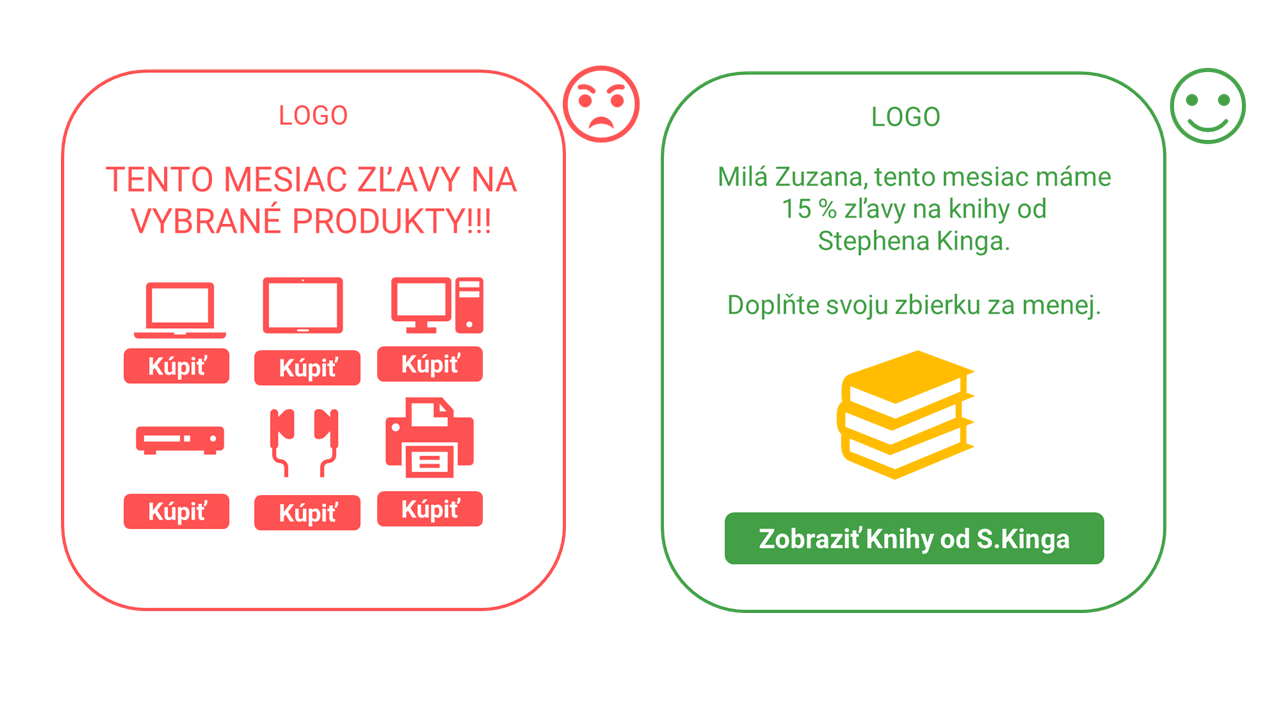The image displays two contrasting sections: on the left, a red box featuring a frowning face emoji, and on the right, a green box with a smiling face emoji. The red box contains text in all capital letters that reads "LOGO TENTO MESSIAH X LA VINA VIBRANAE PRODUCTI," accompanied by clip art graphics depicting various electronic devices such as a laptop, tablet, computer, printer, headphones, and possibly a TV projector or sound system. The green box, labeled with "LOGO NILO ZUZANA TENTA MESSIAH KAME 15%," showcases a clip art graphic of a stack of yellow books. This imagery suggests a comparison between digital and analog modes of information or reading materials, depicted through the respective electronics and books, with the language seemingly indicating diverse product categories.